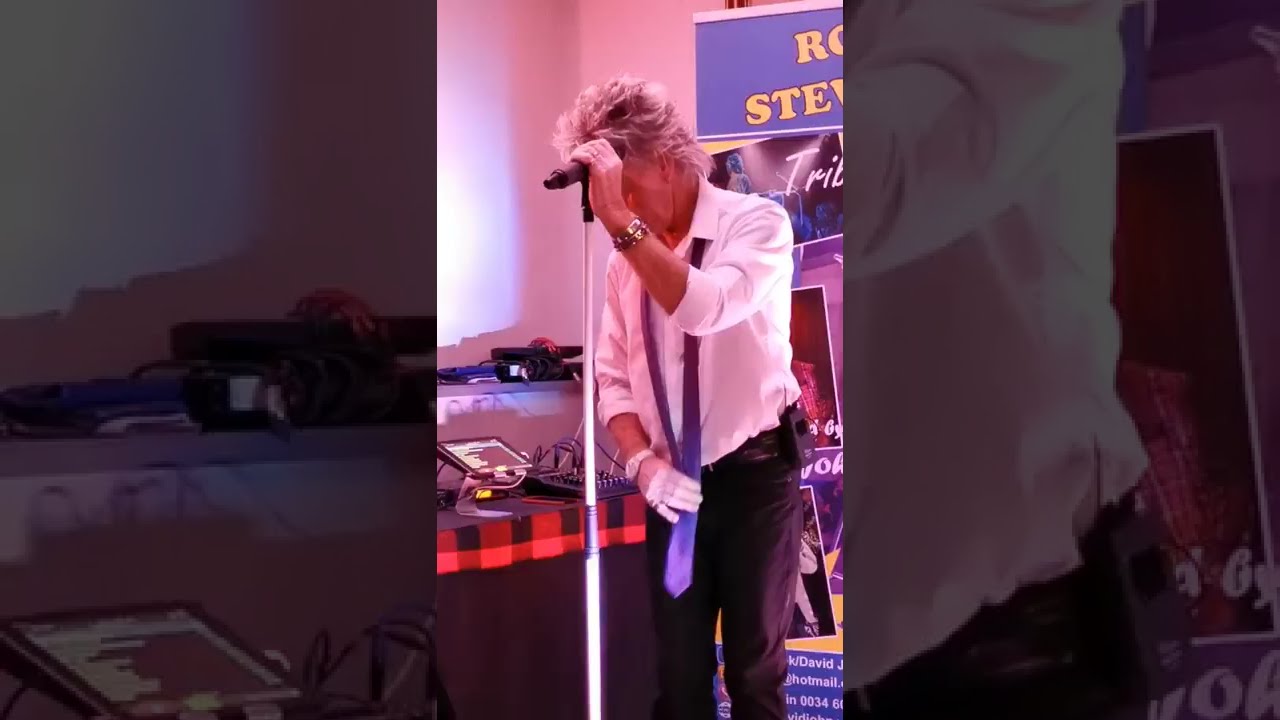This vertical cell phone photo captures a man, likely an impersonator of Rod Stewart, standing at a tall microphone stand with his head down, obscuring his face. The man, sporting characteristic spiky blonde hair akin to Rod Stewart's, is wearing a white dress shirt with the sleeves rolled up to his elbows and a blue tie draped around his neck, untied. He is dressed in dark slacks, with a watch on his right wrist and gold bracelets adorning his left wrist. His left hand grasps the microphone, while his right hand holds the tie at his waist. Behind him, there is a table draped in a black tablecloth with a red buffalo plaid runner, laden with audio equipment and sound boards. In the background, a banner partially shows the letters "R.O." and "S.T.E.," possibly indicating the word "Rod Stewart" or "tribute." The scene suggests he is part of a Rod Stewart tribute act.